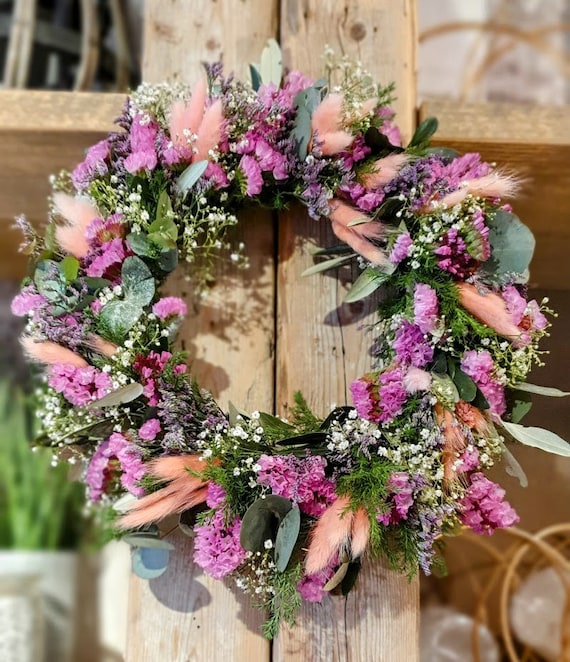The image is a color photograph in portrait orientation showcasing a bright and colorful handmade wreath. The wreath, which hangs on a large wooden post, is adorned with a variety of dried and fresh flowers, including soft pink carnations, clusters of white baby's breath, and small purple floral accents. Delicate, feathery pink-like decorations and light orange feathers add a whimsical touch, while sprigs of green leaves, eucalyptus, and herbs provide lush greenery. The background features out-of-focus, rustic elements with chairs that have wooden backs, hinting at an indoor setting, likely a venue with an upper floor made of thick wood. The overall composition highlights the dainty yet vibrant nature of the wreath, making it suitable for either a wedding or a spring event.